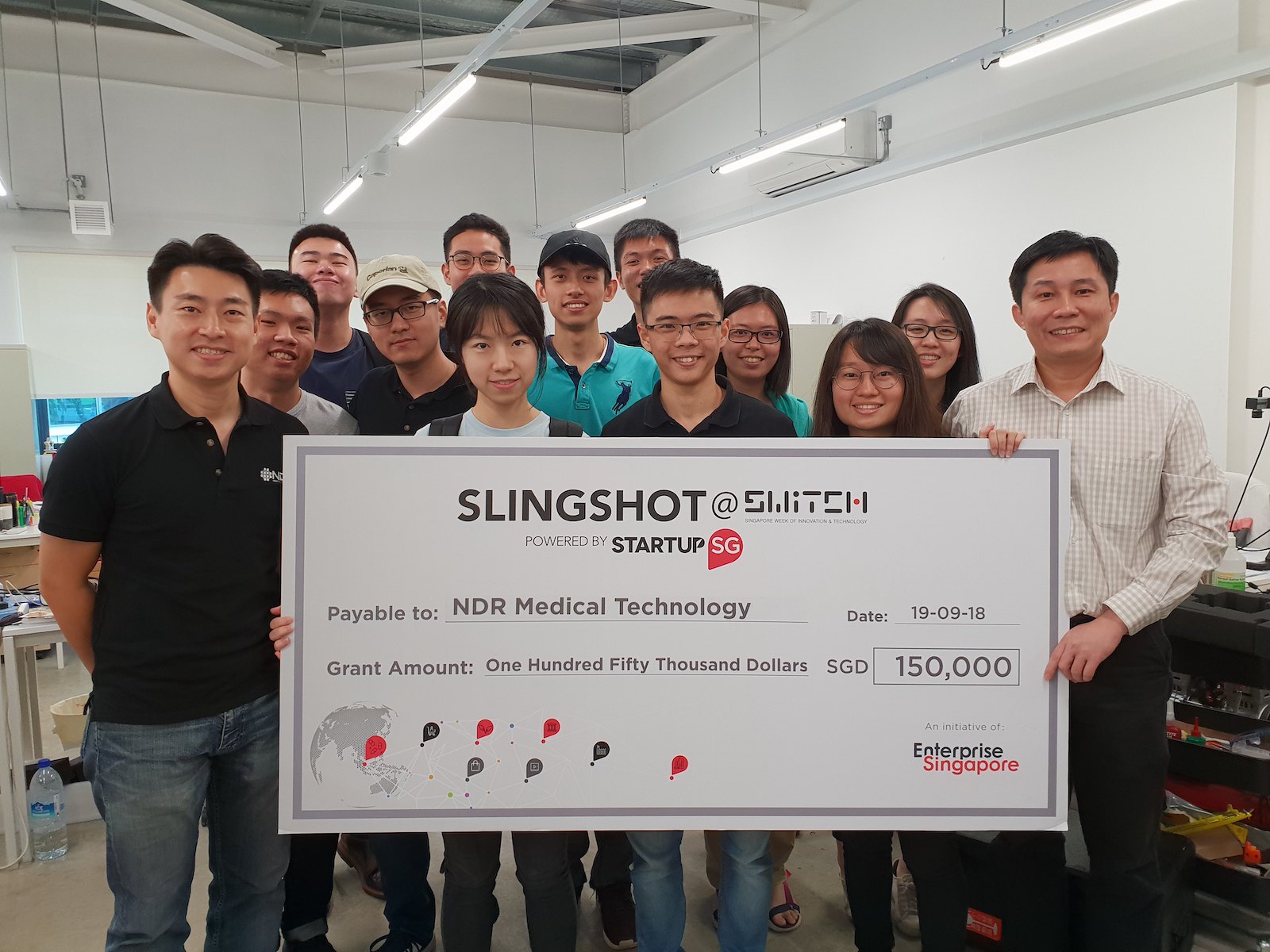This is a detailed indoor photograph featuring a group of approximately 13 to 15 young Asian men and women, predominantly in their 20s to 40s. They are posing with a giant check that reads "Slingshot at Switch powered by Startup SG, payable to NDR Medical Technology" with a grant amount of $150,000, dated 19-09-18, and marked with "Enterprise Singapore" in the bottom right corner. Everyone is smiling and looking at the camera, suggesting a celebratory moment. The group stands in a workshop-like setting with white walls, fluorescent tube lighting, and tables cluttered with equipment and cleaning supplies visible in the background. Notably, a man in a short-sleeved black shirt and blue jeans stands on the left side of the check. Next to him, a young woman with short black hair and overall straps over a light blue shirt is holding the check. There are also other individuals including a man in a brown and white striped shirt, and another man in glasses with a dark top and blue jeans, among others. The atmosphere appears jubilant as they showcase the large check.